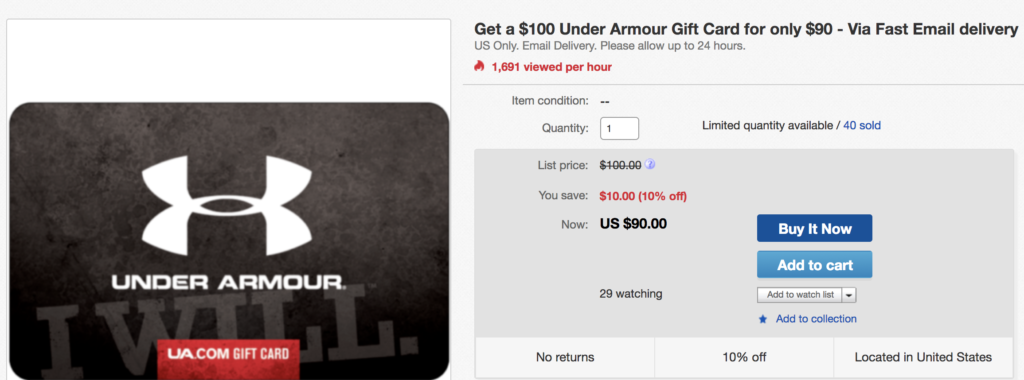This image depicts an online purchase interface for an Under Armour gift card. Dominating the left-hand side of the screen is a gray Under Armour gift card featuring the brand's iconic logo centered above the words "Under Armour." Just below this, the card's background includes the motivational phrase "I Will." Positioned in a red box at the bottom left and center-aligned is the text "UA.com Gift Card."

To the right of the gift card image, there are interactive buttons labeled "Buy It Now" and "Add to Cart." Above these options, a title promotes a special offer: "Get a $100 Under Armour Gift Card for only $90 via fast email delivery." Additionally, the interface indicates that the item has been viewed 1,691 times per hour. The price is prominently displayed as $90, emphasizing a saving of $10, or 10% off the original value.